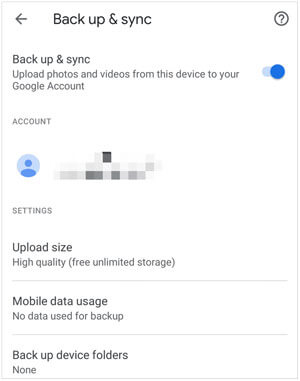This screenshot features a user interface with a clean, white background. Prominently situated in the upper left-hand corner is a gray, left-pointing arrow. To its right, in larger black letters, the text reads "Back up & sync." On the far right edge, there is a circular icon outlined with a black line, containing a black question mark within it.

About five lines down, the phrase "Back up & sync" is repeated in black text. Beneath this, a gray subtext reads, "Upload photos and videos from this device to your Google account," accompanied by a toggle switch on the right. The switch is turned on, indicated by its blue color.

Approximately three lines below, the text "ACCOUNT" appears in gray, all caps. Another three lines down, there is a blue profile icon, styled as a simple circle with a semicircle beneath it. The detailed information to the right of this icon is obscured, represented by gray and black boxes.

Continuing further down, the word "SETTINGS" appears in gray, all caps. Three lines below this, in bolded gray text, is "UPLOAD SIZE." Below this, in smaller gray text, is the line "High quality (free unlimited storage)" followed by a light gray horizontal divider.

Further down, the bolded gray text "MOBILE DATA USAGE" is visible, under which it states in gray text "No data use for backup," followed by another light gray horizontal line.

Towards the bottom, the section titled "BACKUP DEVICE FOLDERS" is noted in bolded gray text. Underneath this heading, the word "None" is displayed in gray.